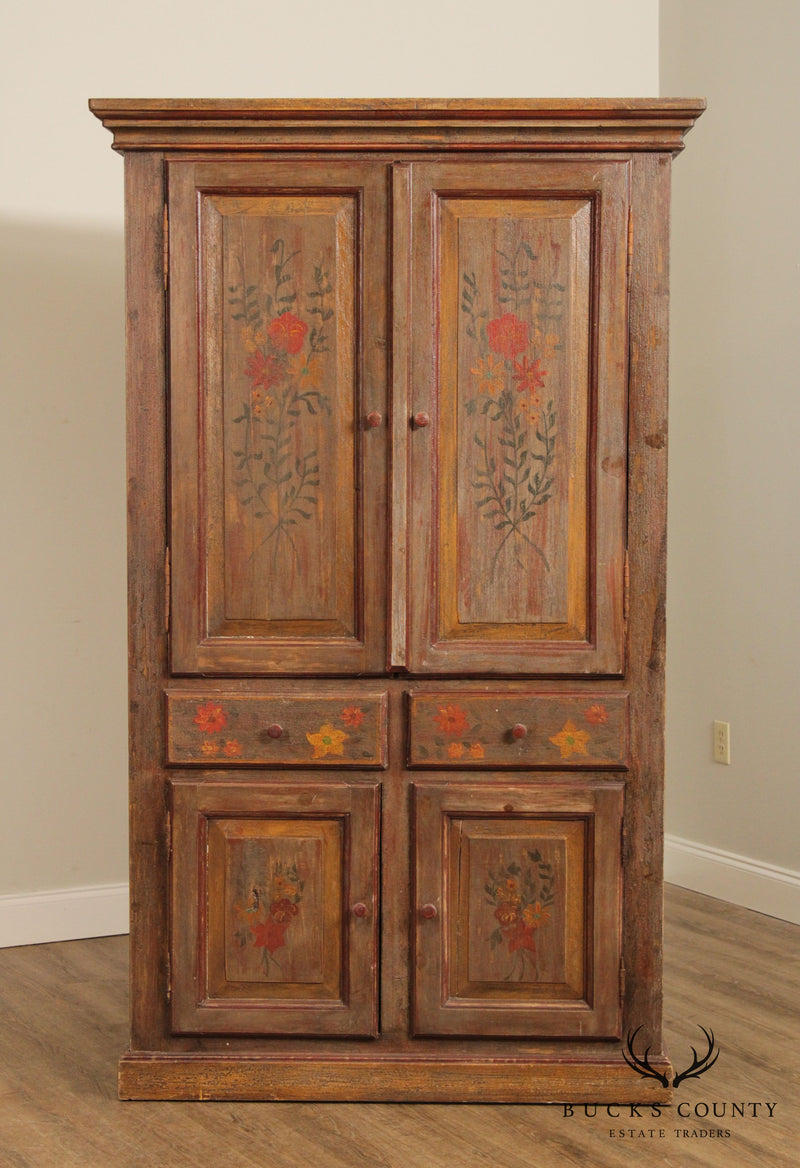This image portrays a large, antique wooden cabinet standing on a wood floor against a tannish background wall. Highlighted by good lighting that casts a slight shadow, the cabinet is a lighter brown color and showcases signs of wear, particularly at the bottom. The cabinet features two tall, vertical doors with round wooden knobs on top, two small matching drawers beneath, adorned with orange and yellow flowers, and two smaller vertical doors at the bottom, also with round knobs and painted with vibrant flowers and green leaves. The floral designs on the cabinet, which include red and yellow flowers, appear hand-painted and suggest either an amateur or aged craftsmanship, adding to its antique charm. In the bottom right corner, the image includes the logo of Bucks County Estate Traders, depicting black antlers. An electrical socket is visible to the right of the cabinet, further detailing the setting.